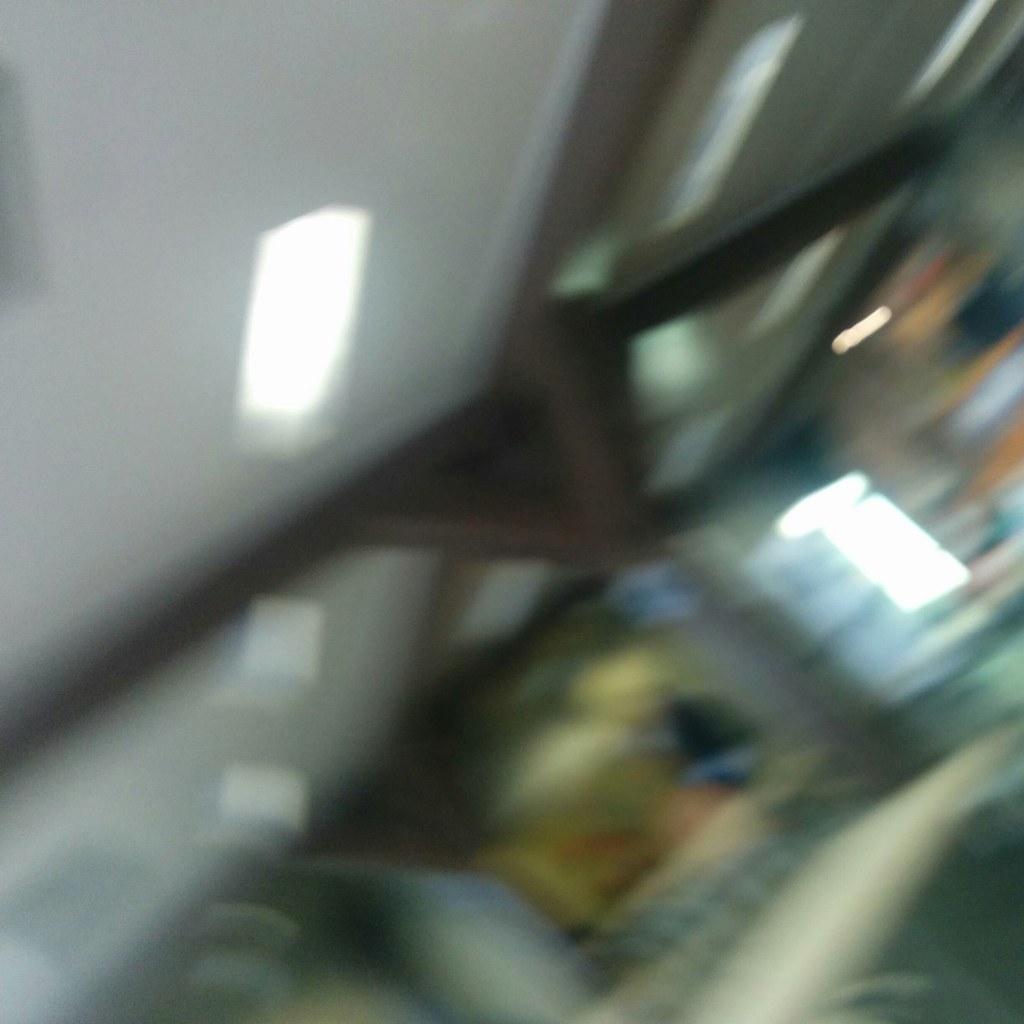This indoor photo, taken at an unusual angle, is quite blurry. The image features a predominantly white surface, running along the left side with three illuminated shapes – a rectangle and two squares. From left to right, a brown rod or beam extends across the frame, with a V-shaped brown section rising upwards. A bright light is located on the right side of the image. The photo exhibits a gradient of colors, transitioning from yellow in the middle to orange and blue towards the bottom. Additionally, a structure resembling an arm protrudes from the bottom, while the right side displays patches of orange and the upper right corner is illuminated.